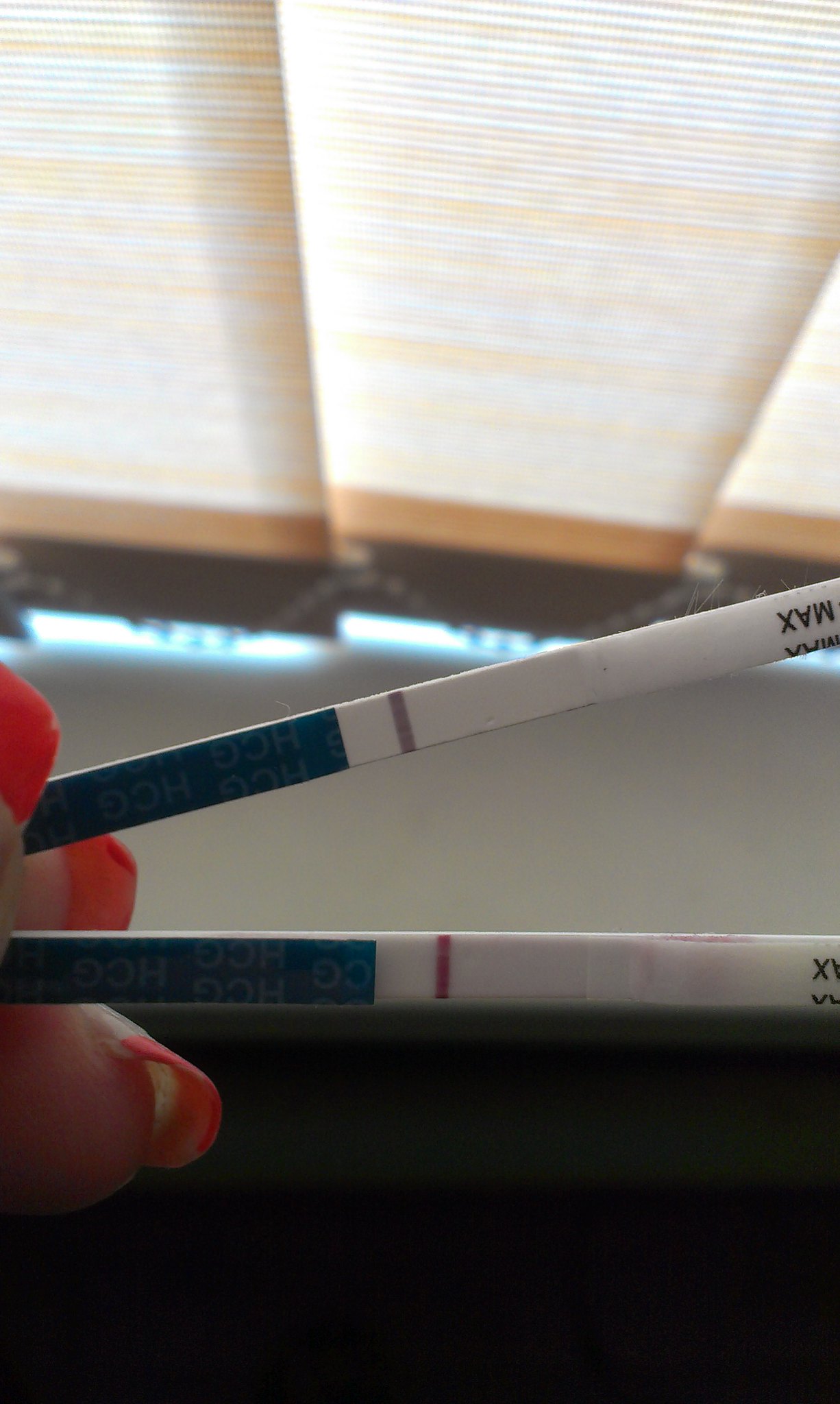The image shows a close-up of a person's hand holding two pregnancy tests. One test is positioned horizontally, while the other test is angled from the left side upwards to the right. The background reveals a partially visible, striped curtain with colors that include yellow, orange, and blue, descending approximately halfway down the image. Below the curtain, there's a thicker orange border followed by a thicker black border. 

In the area where the curtain ends, light illuminates a white wall that extends down about a third of the image's height. Overlapping parts of the image, similar to a collage, show another section of the curtain against a white wall and a green border approximately one-third down the image, followed by black. 

A fingertip with a yellow nail and an orange tip is visible near the green border. Between the two pregnancy tests, there is a partial view of another fingertip with an orange-tip fingernail. An orange-tinged thumb helps hold the top test from the left side. 

The horizontal pregnancy test has a blue section with "HGC" written in lighter lettering, followed by a white square and a red vertical stripe. The rest of the test is white with some black lettering towards the end. The second test, following the same design, features "max" in black letters near its end.